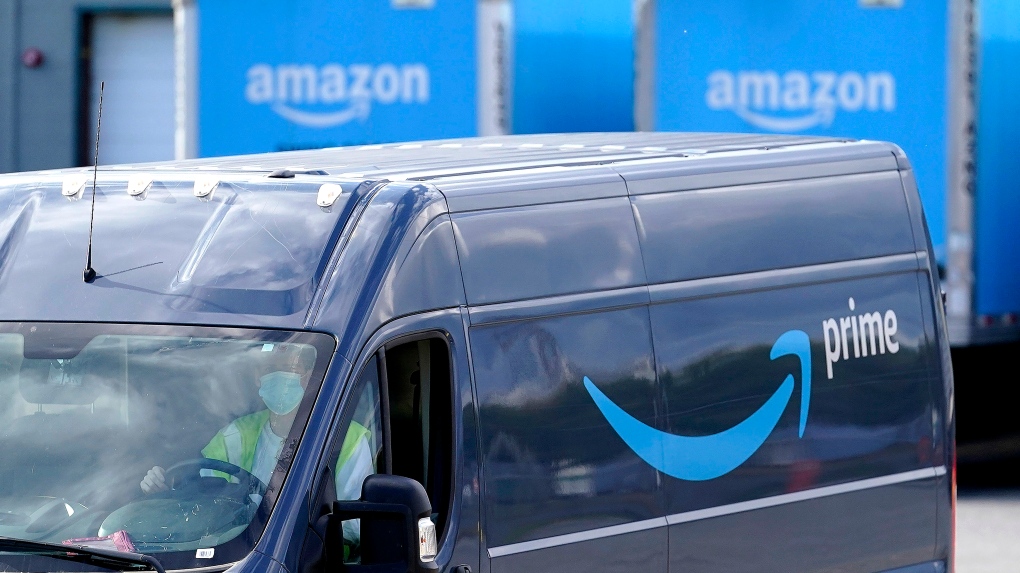The photograph portrays an Amazon loading bay set outdoors on a sunny day. In the background, a lineup of blue Amazon trucks are neatly parked, each emblazoned with the distinctive Amazon logo. Dominating the foreground is a dark blue Amazon Prime van, its driver's side window rolled down. The van prominently features the familiar light blue arrow and the word "Prime" in white on its side. 

Inside the van, a driver is discernible, clad in a high-visibility jacket and a face mask covering their mouth and nose, with hands firmly grasping the steering wheel. A small antenna is visible on the van's front. Although the lower portion of the photograph is cropped, an intriguing reflection on the side of the van hints at the environment. The reflective metal surface captures the image of green trees and a predominantly blue sky dotted with a few clouds, suggesting a bright and clear day.